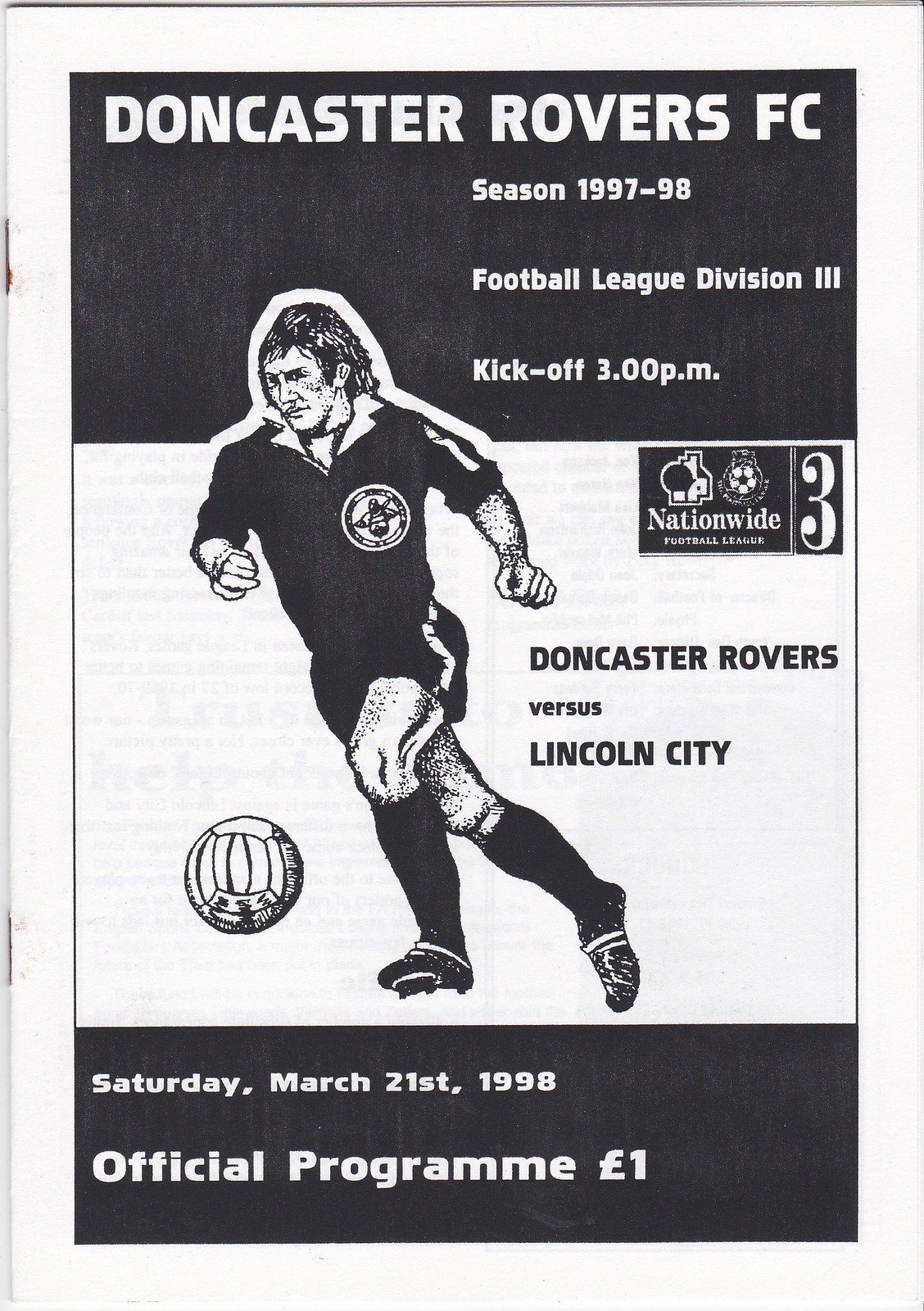The image features the cover of an official program for a football match. Dominated by black, white, and a hint of gray, the cover showcases an image of a soccer player at its center, captured mid-action as he kicks a ball. The soccer player is attired in a traditional short-sleeved, collared uniform complete with shorts. Above this dynamic illustration, bold white text announces:

"Doncaster Rovers FC
Season 1997-98
Football League Division 3
Kickoff 3 p.m."

Further details indicate the match specifics:
"Doncaster Rovers vs. Lincoln City
Saturday, March 21, 1998
Official Program
£1.00"

This program book, traditionally provided to spectators upon entering the stadium, encapsulates the event's details in a visually engaging manner.